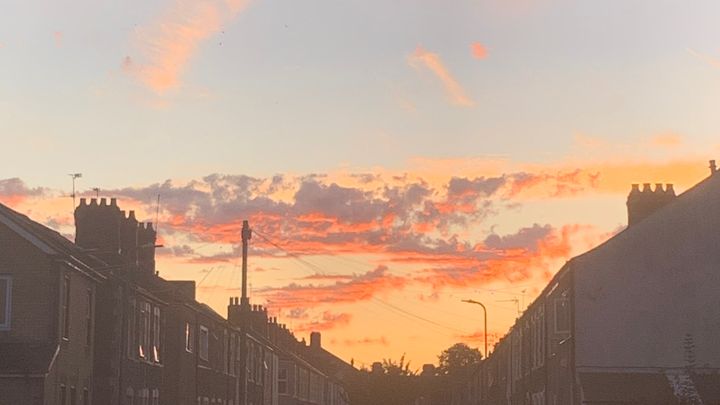This color photograph captures a city street at either sunrise or sunset, with a washed-out, slightly overexposed quality. The sky at the top is mostly a pale blue, transitioning into a sea of scattered billowing clouds lit from below in vibrant hues of orange, yellow, pink, purple, and gray. The scene is framed by rows of beige and brown row houses or townhouses on both sides of the street, which are only visible from the top of the first-floor windows upwards. Attached buildings recede into the distance, giving the impression of perspective narrowing towards the center. Some buildings feature chimneys resembling castle towers, and most have multiple windows, though details are faint due to the lighting conditions. Streetlights and telephone poles with wires stretch across the scene, adding a touch of urban infrastructure. While the image captures the serene, colorful sky and the architectural elements, it is devoid of people, animals, and moving vehicles, focusing solely on the tranquil moment in the city.